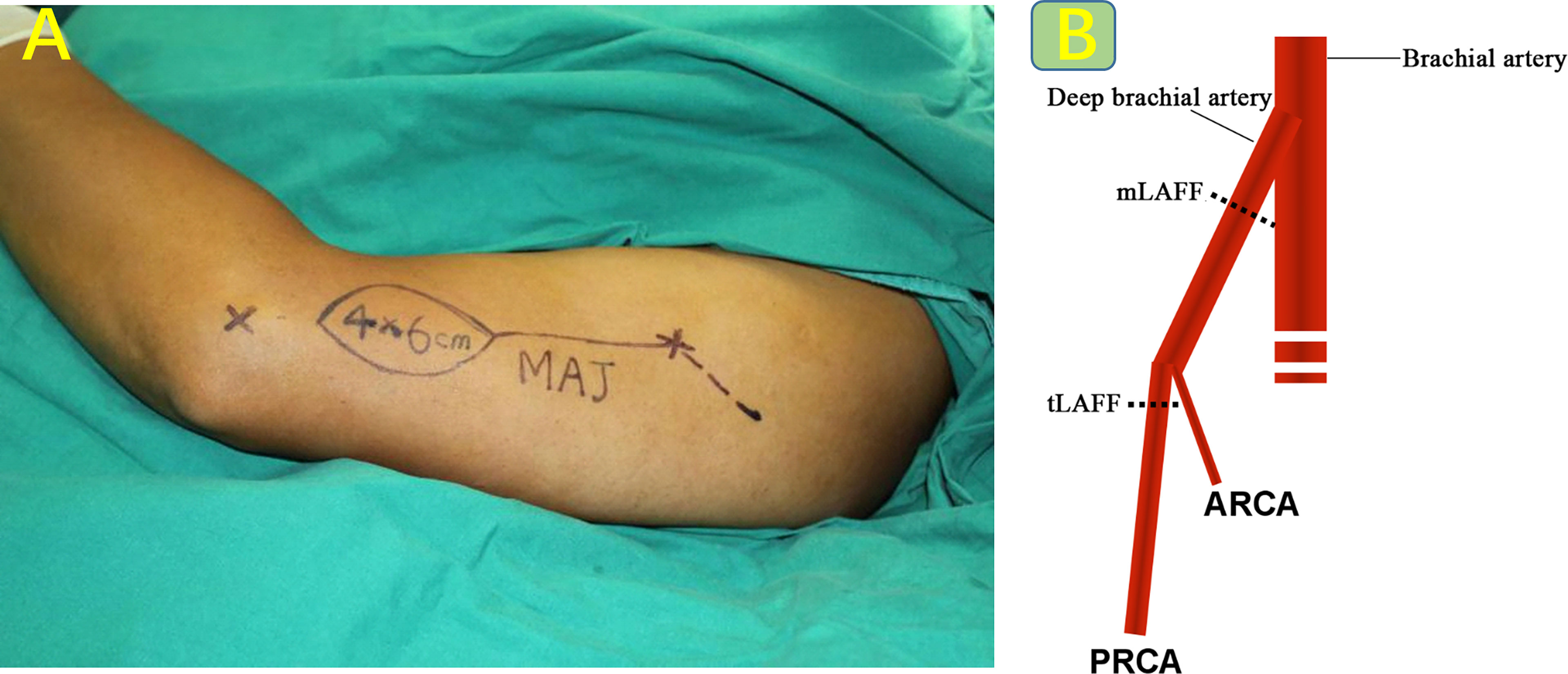The composite image consists of two distinct sections, positioned side by side. The top of the image features labels indicating 'A' on the left and 'B' on the right.

**Left Section (A):** This section displays an image of an individual's arm showcasing a medical marking. The marking is prominently black in color and has an oval-shaped boundary. Inside this oval, the dimensions "4 x 6 cm" are inscribed. Additionally, the marking bears the letters "M A J," possibly indicating a medical annotation or identification code.

**Right Section (B):** This section features a detailed medical diagram illustrating the vascular anatomy of the arm. The diagram highlights various arteries in red, meticulously labeled to indicate different parts. Key labels include the brachial artery, deep brachial artery, medial antebrachial (MLA), lateral antebrachial (TLA), anterior radial collateral artery (ARCA), and posterior radial collateral artery (PRCA).